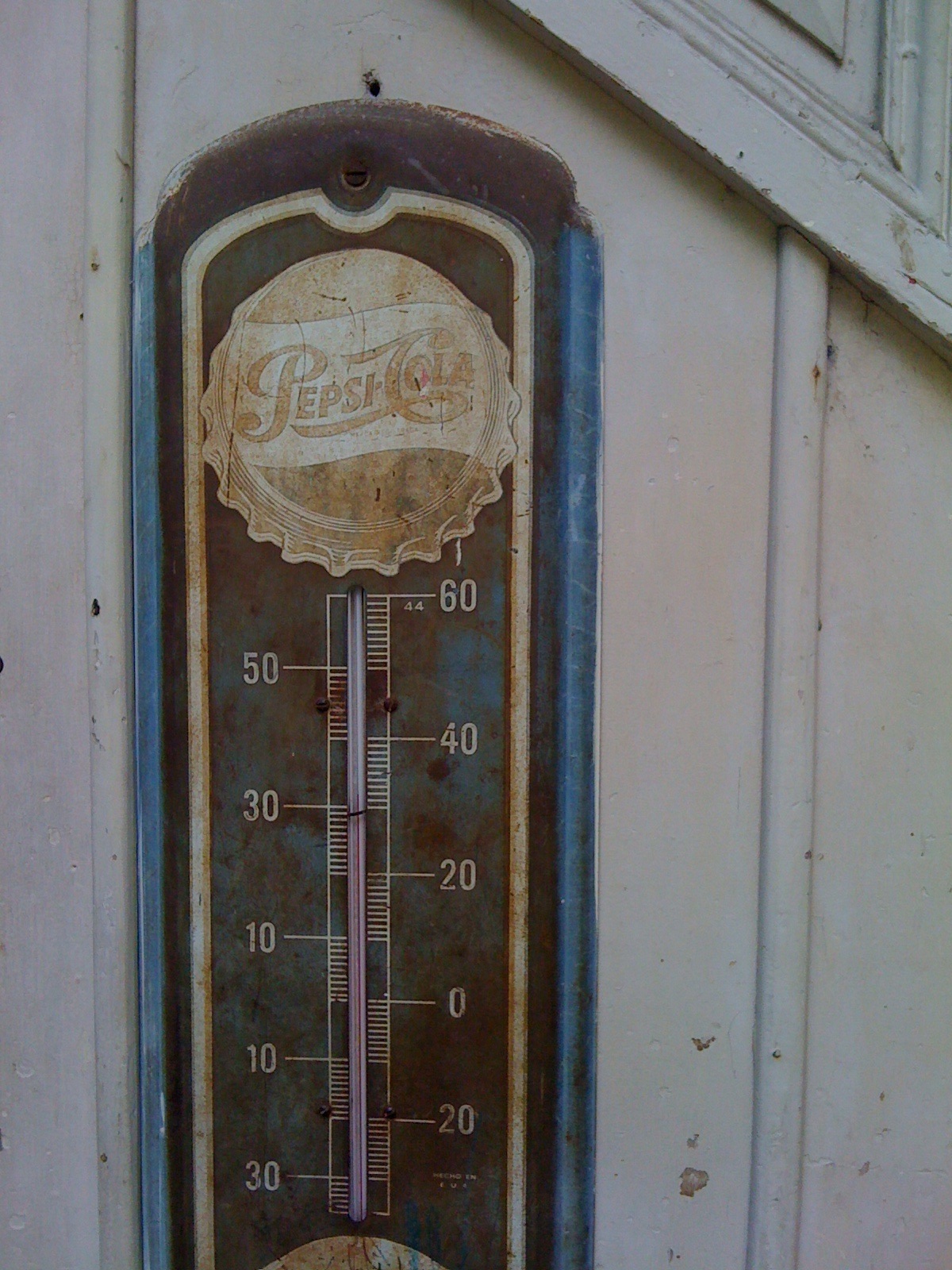The photograph showcases a vintage Pepsi Cola thermometer mounted against an aged, white wooden wall. The thermometer, which stands vertically, features a predominantly brown and gray color scheme with hints of faded blue along the sides. The Pepsi Cola logo, located in the center, is heavily faded to an almost white hue, indicating the item's considerable age. The numbers for the temperature readings are displayed in descending order from 60 at the top to -30 at the bottom, marked at intervals of 10 degrees (60, 50, 40, 30, 20, 10, 0, -10, -20, -30). The numbers are connected to a clear tubing that runs down the middle of the thermometer, likely indicating the temperature. The overall condition of both the thermometer and the wooden wall behind it suggests significant wear and weathering, adding to the vintage charm of the scene. The composition is tightly framed, making it difficult to ascertain the exact size of the thermometer, but it remains the focal point of the image.